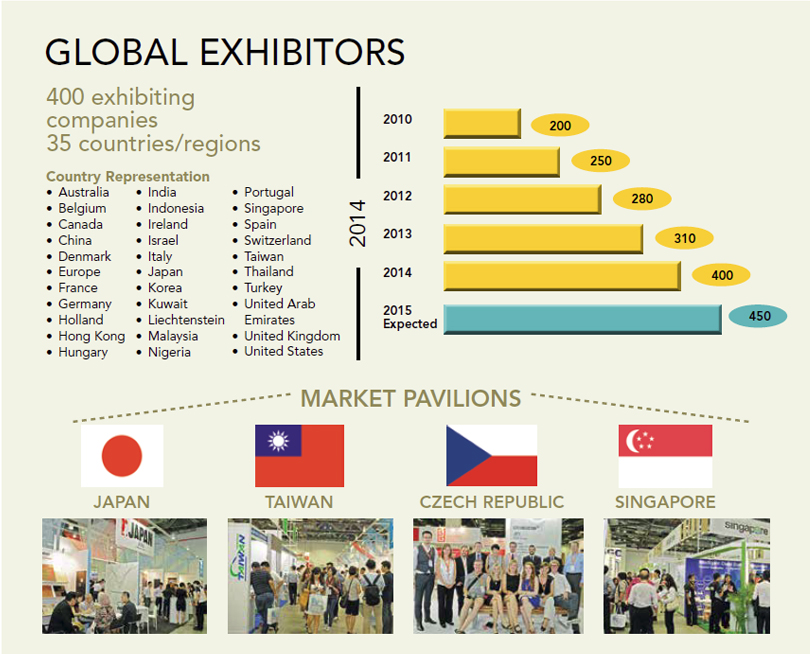This infographic, outlined on a pale white-yellow background, provides a detailed overview of global exhibitors. In the upper left corner, "Global Exhibitors" is prominently displayed in black, followed by the text "400 exhibiting companies from 35 countries/regions." Below, a three-column bulleted list denotes country representation, including Australia, Belgium, Canada, the United States, the United Kingdom, Japan, and Italy, in alphabetical order.

To the right, a line graph with horizontal yellow bars, turning light green in 2015, showcases growth from 2010 to 2015 (expected). The bars indicate numerical values: 2010 at 200, 2011 at 250, 2012 at 280, 2013 at 310, 2014 at 400, and 2015 at 450. Above the graph in black text, it reads "Global Exhibitors" and "400 exhibiting companies, 25 countries/regions."

At the bottom center, under the heading "Market Pavilions" in gold, flags of Japan, Taiwan, the Czech Republic, and Singapore are displayed, each labeled with their respective country names. Beneath each flag, thumbnail images depict crowds gathered at these market pavilions.